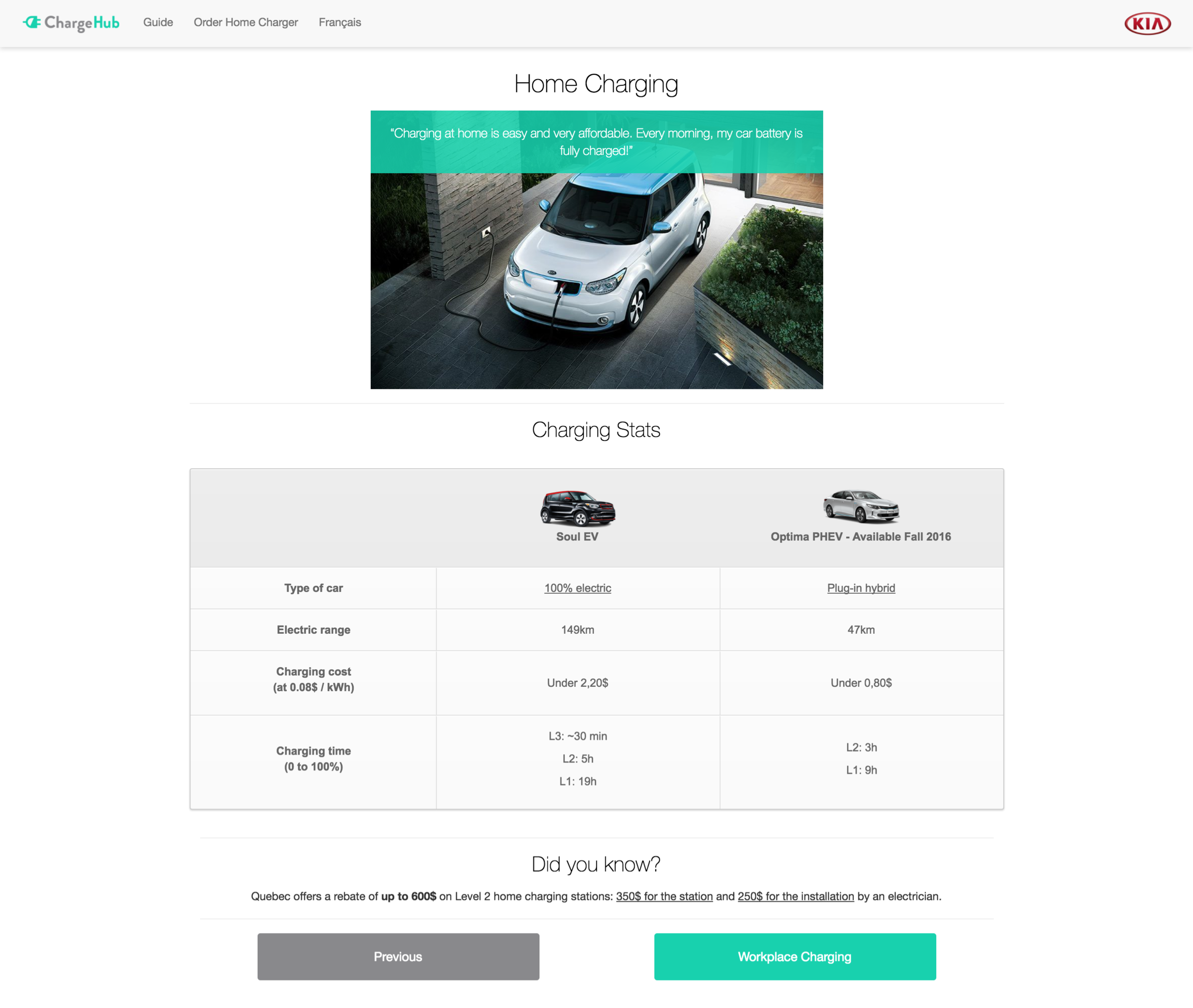Here is a detailed and cleaned-up caption for the image:

---

This image showcases a website dedicated to guiding users on home electric vehicle (EV) chargers. The webpage is titled "Charge Hub Guide: Order Home Charger and Franchise." It emphasizes the ease and affordability of home charging, stating that charging at home is convenient and budget-friendly. A personal anecdote notes that the car's battery is fully charged every morning. The image also features a small car connected to a charging cable, visually representing the home charging process. Additionally, there is a table that provides charging statistics, including columns for the type of car, electric range, charging cost, and charging time, with detailed information listed under each category.

---

This caption is thorough and highlights all the key elements depicted in the image.